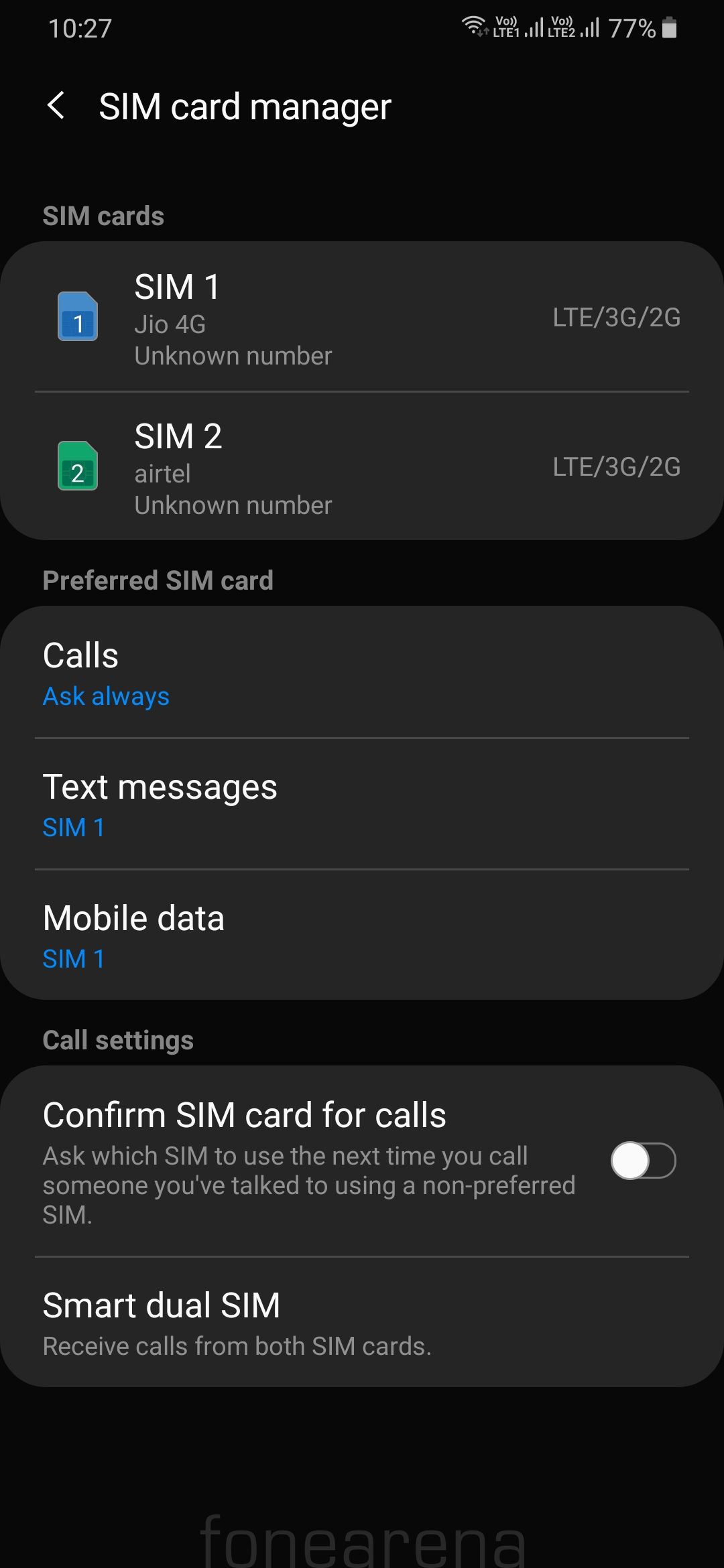Screenshot depicting a SIM card management interface on a device, set against a black background, with a battery level displayed at 77%. The device model indicated is "Tom 1027". 

The interface shows two SIM cards labeled as:
- **SIM 1**: Marked with a number "1" in a blue square, supporting LTE/3G/2G networks.
- **SIM 2**: Marked with a number "2" in a green square, also supporting LTE/3G/2G networks.

Under the "Preferred SIM card" section, three gray rectangles categorize the preferred functions, with the following settings:
- **Calls**: Default app is always highlighted in blue.
- **Text messages**: Set to SIM 1 and highlighted in blue.
- **Mobile data**: Also set to SIM 1 and highlighted in blue.

Under "Call settings", the interface includes:
- **Confirm SIM card for calls**: Option to ask which SIM to use the next time you call someone you have previously contacted using a non-preferred SIM. This setting is currently toggled off.
- **Smart Dual SIM**: Feature to receive calls from both SIM cards.

At the bottom of the screenshot, the source "Phone Arena" is mentioned.